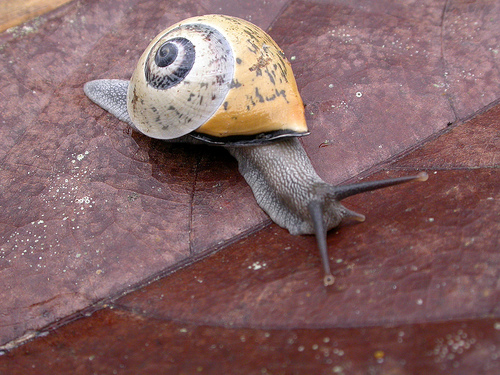This detailed image captures the intriguing journey of a large snail moving across a diagonal divide of a brown, stone-like surface, which appears wet on one side. The surface hosts a fascinating contrast: a darker, possibly moist area, set against a lighter brown section, hinting at its stone texture. At the very center of the composition, the grayish, textured snail, adorned with white bumps, takes prominence. Its two extended antennae, crowned with circular ends, lead the way as it plants its face firmly on the ground, seemingly exploring its surroundings with intent.

The snail's shell is a striking visual feature: predominantly yellowish-gold with black speckles and a softer gray spiral pattern that fades outward from a black center. The shell’s dynamic coloration and spiral design are echoed in the delicate interplay of light and shadow on the shell's surface.

This close-up nature photograph highlights the snail's intricate details, from its textured body to its towering shell, against a backdrop that juxtaposes wet and dry textures, emphasizing the snail's tranquil, yet purposeful crawl across the stone plane.